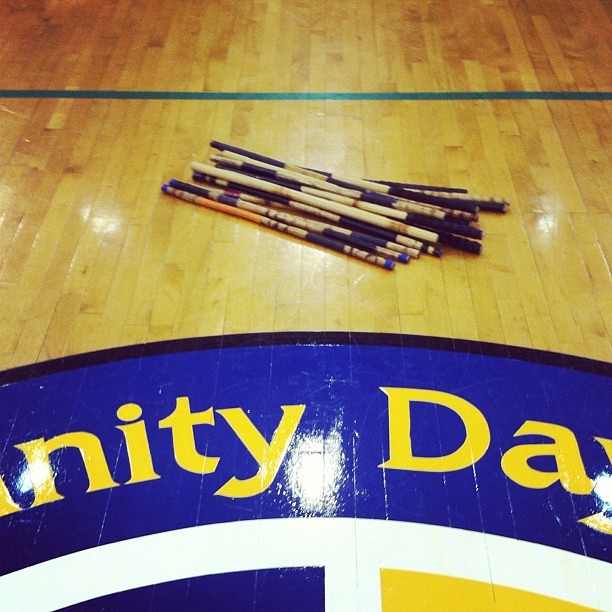This photograph depicts a shiny brown wooden floor, likely part of a gymnasium. At the center, partially cropped, there is a blue semicircular graphic with a thin black border and an inner white line. In this graphic, the letters “N-I-T-Y D-A” are visible in yellow, hinting at the phrase “Unity Day.” Flanking the white line are blue and yellow segments, suggesting school colors. Near the top, a blue line crosses the floor, indicating a division for a sports court. Lying across the floor are approximately ten wooden sticks, each about a couple of feet long, with dark blue tape wrapped around them and some possessing blue, light blue, or even orange tips, resembling pool cues with chalked ends.